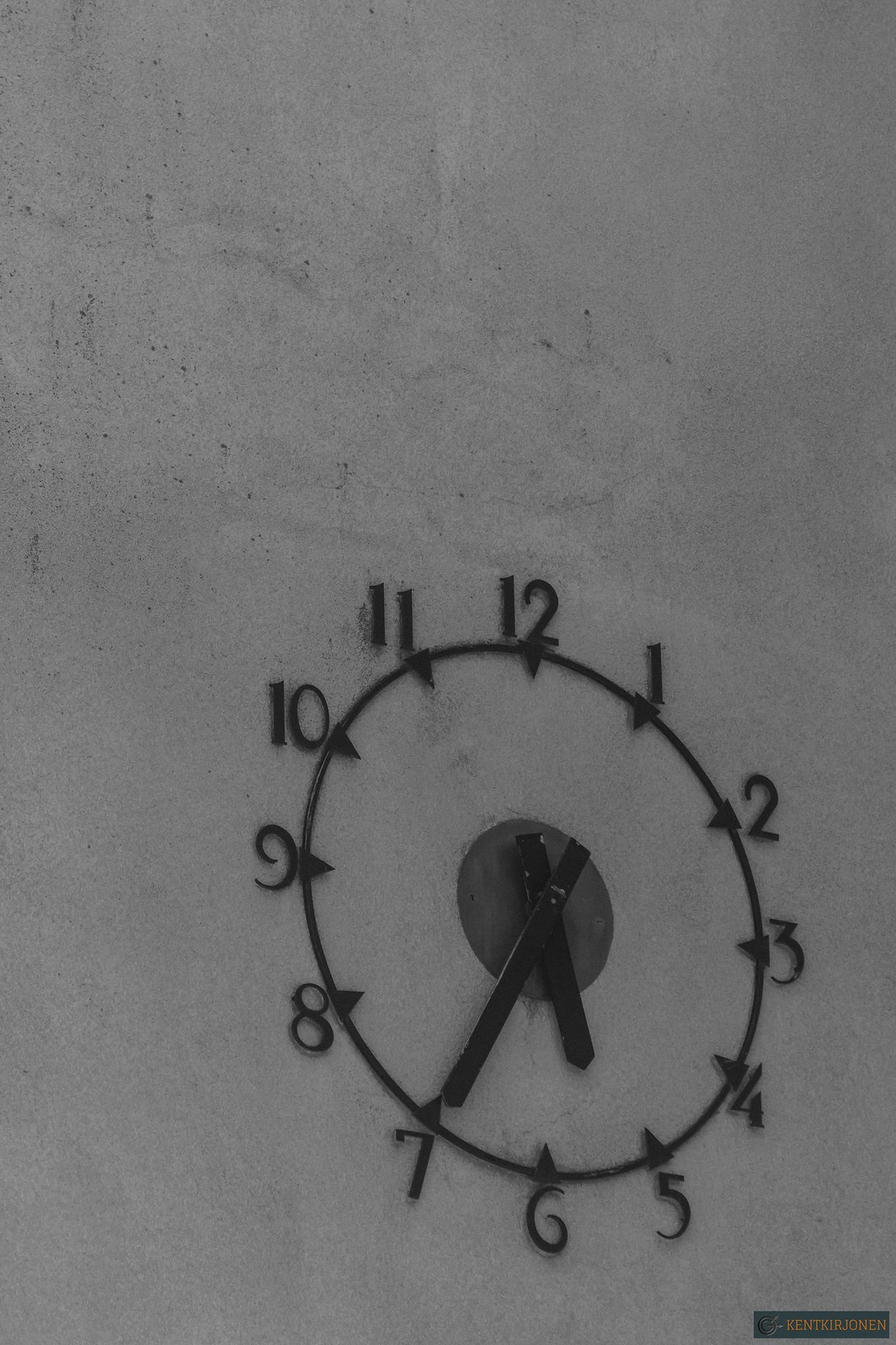The photograph features a large, minimalist clock mounted on a grayish-white concrete wall. The clock is composed entirely of exposed black metal, giving it a skeleton-like appearance with no glass or exterior casing. The clock starts towards the bottom right-hand corner of the dark image, where a small, rectangular black object is pointing. The outer rim of the clock displays the numbers 1 through 12 in a clockwise direction, each affixed directly to the wall. In the center of the clock, a smaller circle holds the black metal hands, which indicate the time as 5:35. The photograph is stark and simplistic, capturing only a portion of the rugged concrete wall, adding to the industrial aesthetic of the scene.